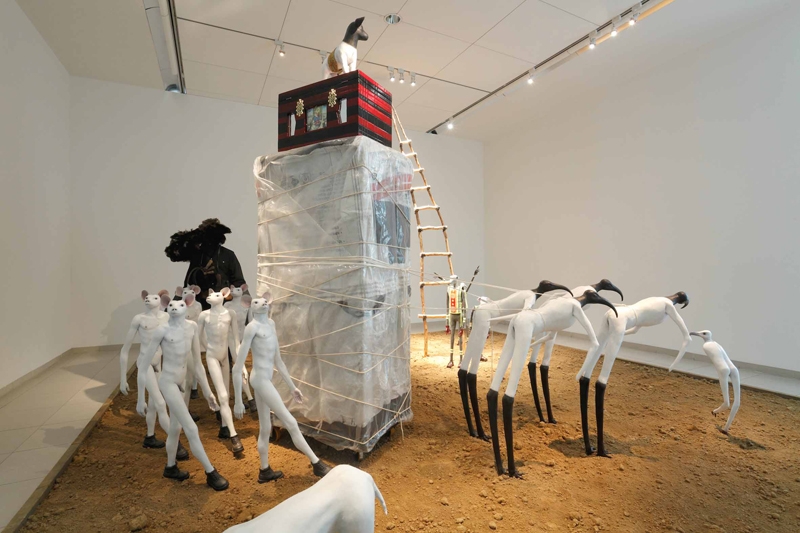The image depicts a surreal and elaborate art installation in a modern art gallery. The gallery features pristine white walls and ceilings illuminated by track lighting. The floor of the installation area is a combination of white tiles and a central rectangular pit filled with brown, dry earth.

At the center of the installation is a towering structure formed from two high-stacked boxes wrapped in clear plastic and bound with string. Atop these boxes sits a red and black striped trunk. Perched on this trunk is a hybrid creature with the body of a sheep and a black head. A ladder extends from the trunk down to the ground, where a sage green humanoid figure with four arms, featuring a prominent '8' penny, stands waiting.

To the left of the installation, five uncanny, white, nude humanoid rats wearing black sneakers are depicted in a marching formation towards a large, ominous black figure with indistinct features in the background. These humanoid rats are anatomically detailed and strikingly surreal.

On the right, humanoid figures resembling birds, with black legs and heads featuring long, elongated beaks, are bent at the waist as if pulling the tower's boxes with ropes. One of these bird-humanoids, entirely white and without wings, displays a human-like buttock definition.

The overall effect of the scene is a bizarre and intricate tableau, blending elements of human and animal forms in an eerily lifelike manner, all set against the sterile and stark backdrop of the gallery's white interior.